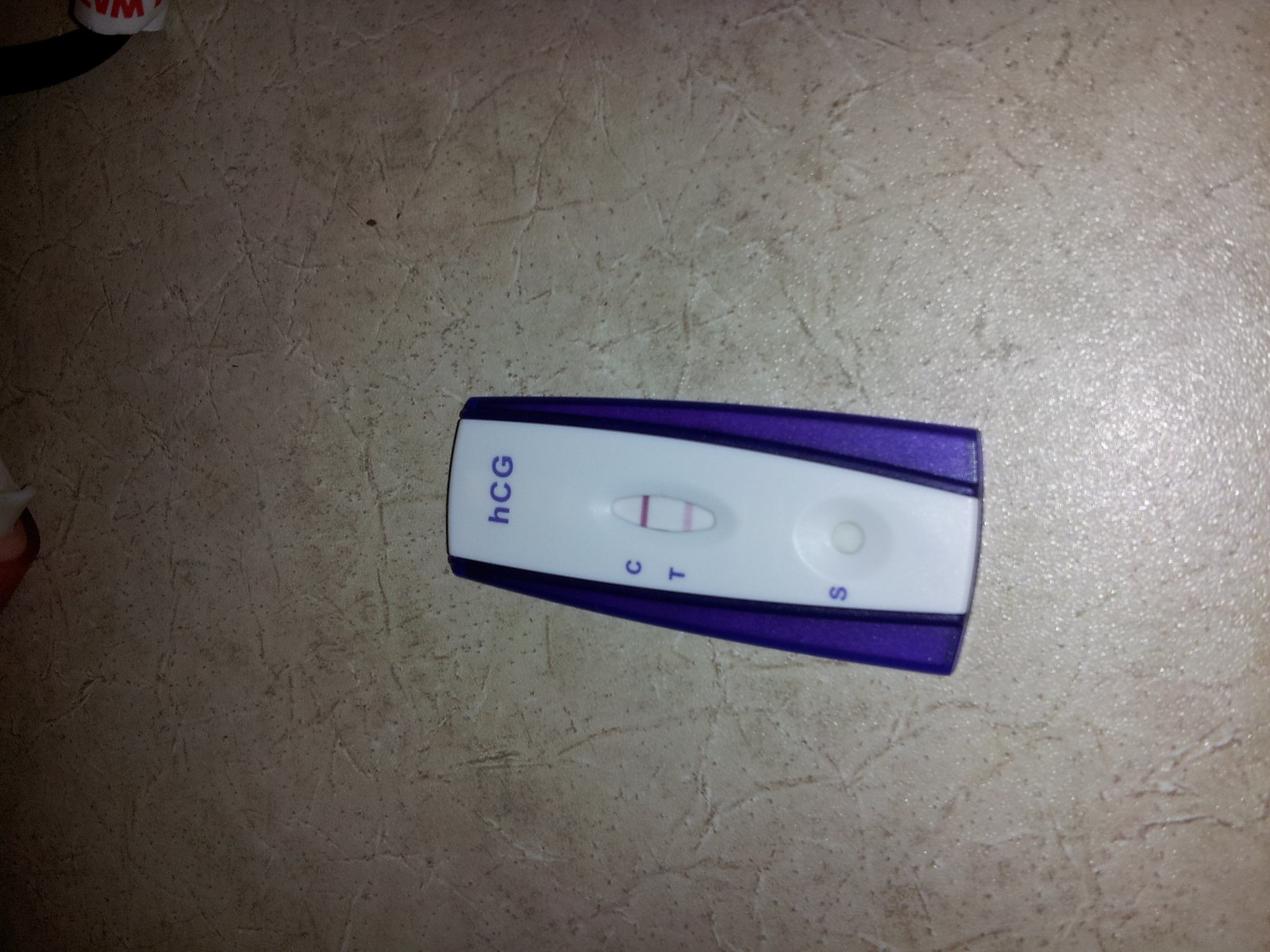In the center of the photograph, a rectangular plastic pregnancy test is prominently displayed. The pregnancy test, bordered in purple with a white center, is oriented diagonally with its top facing the left side of the image and its bottom towards the right. Within the central white area, "hCG" is inscribed, indicating the test's function. Below this inscription is an oval indentation that houses a white piece of paper, featuring a dark purple line at the top and a light purple line at the bottom. The dark purple line is labeled with a capital "C," signifying the control indicator, while the light purple line is labeled with a capital "T," denoting the test indicator. Further down to the right on the pregnancy test, there's a circular indentation with another white piece of paper, adjacent to which is a capital "S" in purple.

The pregnancy test rests on a textured gray floor composed of numerous dark and light gray lines, adding depth to the background. In the top left corner of the photograph, a roll of paper marked with a large red "M" is partially visible, adding an additional element to the composition.